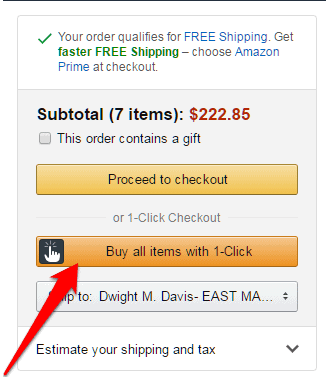Here's a detailed and cleaned-up caption for the given image description:

---

This image captures an Amazon checkout screen, formatted in portrait orientation. The photo appears to be a screenshot from a mobile device or a computer. 

At the top of the screen is a thin black line set against a white background. Below this, a white section contains a thin gray-bordered box. The box is divided by another thin gray line. Within the white background at the top of the box, there's a green checkmark on the left, followed by the text "Your order qualifies for FREE Shipping." The term "FREE Shipping" is highlighted in blue. 

Next, it states, "Get faster FREE shipping," with the phrase "faster FREE shipping" highlighted in green. It then suggests, "Choose Amazon Prime at checkout," with "Amazon Prime" in bold.

Below the dividing gray line, another gray box displays a black font message: "Subtotal (7 items):" accompanied by a price in red - "$222.85." 

An empty checkbox follows, labeled "This order contains a gift." Below this, a long, yellow rectangular button with black text says "Proceed to checkout." Underneath, it offers another option in gray text: "or 1-Click Checkout."

Further down, an orange box with an index finger icon, surrounded by a star, reads "Buy all items with 1-Click." This orange button features black font.

Towards the bottom, "Ship to:" is displayed against a white background with black text, specifying "Dwight M. Davis, East MA." The screen concludes with the option to "Estimate your shipping."

---

This caption provides a detailed and structured description of the image, ensuring clarity and thoroughness.